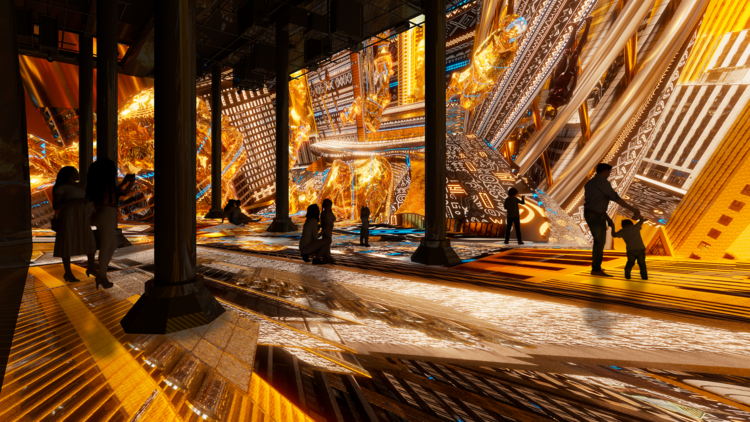The image depicts an immersive art installation inside a building, where the atmosphere is predominantly dark, casting the attendees as shadowy figures. Illuminated walls and floors are adorned with vibrant, artistic projections in shades of gold, blue, white, and brown, displaying a myriad of shapes such as triangles, squares, and rectangles. Some areas appear to mimic the flow of lava. The industrial setup includes shadowed columns supporting an overhead floor, adding to the surreal environment. Attendees, who appear to be of all ages, are seen engaging with the art—some closely examining and even touching the glowing projections, suggesting a sense of wonder and interaction with the dynamic, digitally-created artwork.